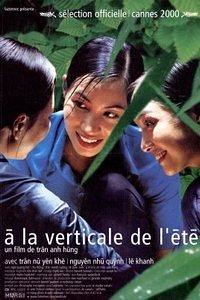The image is a poster of the movie "À la Verticale de l'Été," prominently featuring three young Asian women with black hair tied back in ponytails. They are smiling at each other, dressed in blue shirts that accentuate their features. Their lips are red, adding a striking contrast to their appearance. The background appears lush with green foliage, including both round leaves and long, thin, straight ones that even cascade across the front edges of their faces, suggesting a jungle or garden setting. Text on the poster, presented in French, includes "Sélection Officielle Cannes 2000" at the top, indicating the film was an official selection at the 2000 Cannes Film Festival. Additional text is present but mostly unreadable due to blurriness or language barriers.